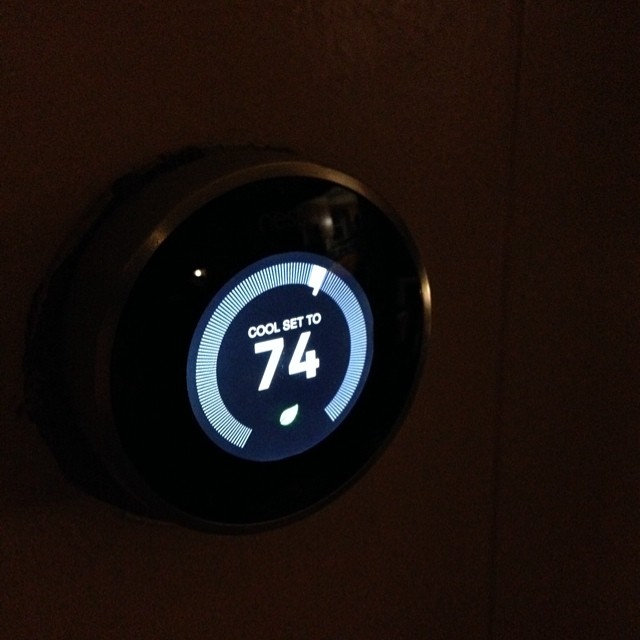This image captures a Nest Thermostat displaying a cooling setting of 74°F against a dark background. The thermostat features a sleek, circular design with an embedded digital display. A series of blue tick marks form a ring around the perimeter of the display, gradually transitioning into a white gradient for a modern, polished look. A tiny, thumbtack-like light glows subtly, adding a touch of elegance to the device. Positioned below the temperature reading, a small green leaf icon, rendered in white, signifies the energy-saving mode of the thermostat.